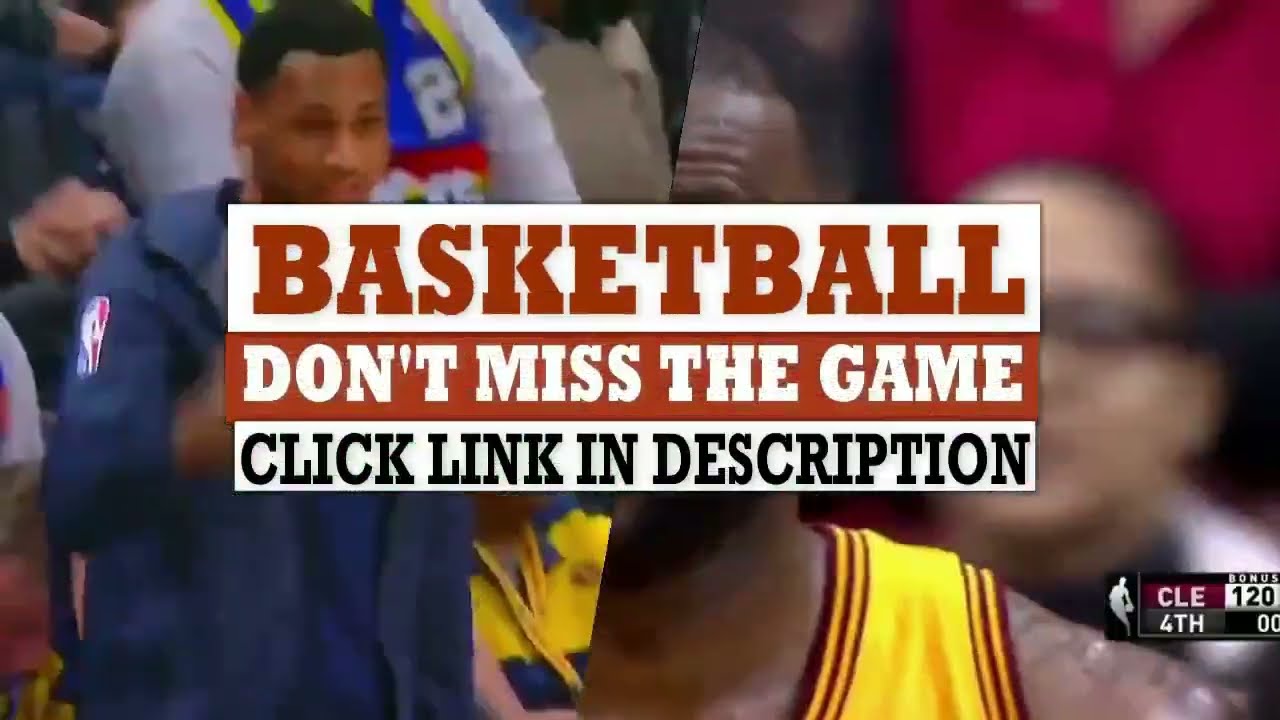In this image, the central focus is a promotional banner urging viewers to click a link in the description for more details about a basketball game. The banner prominently displays the word "Basketball" in bold, dark orange letters on a white rectangular background, beneath which it says "Don't miss the game" in white letters against a dark orange backdrop. Directly under this, the text "click link in description" is showcased in black letters on a white background, all using a sporty serif font in capital letters. 

On the left side of the image, there's an African American man wearing a navy blue jacket emblazoned with the NBA logo on the sleeve, likely indicating an official or staff member. Behind him, the blurred outline of a crowd suggests the presence of fans in a stadium. To the right, part of another African American individual is visible; he is donned in a yellow basketball jersey with maroon accents, likely a player. 

Amidst this scene, overlaying the background, is a partially obscured scoreboard stating "Cleveland" and indicating a score of 120 and that it's the fourth quarter, although details about the opposing team and the exact time remaining are not visible. The overall composition of the image strongly emphasizes an invitation to not miss out on the basketball game and to engage further by clicking the provided link.